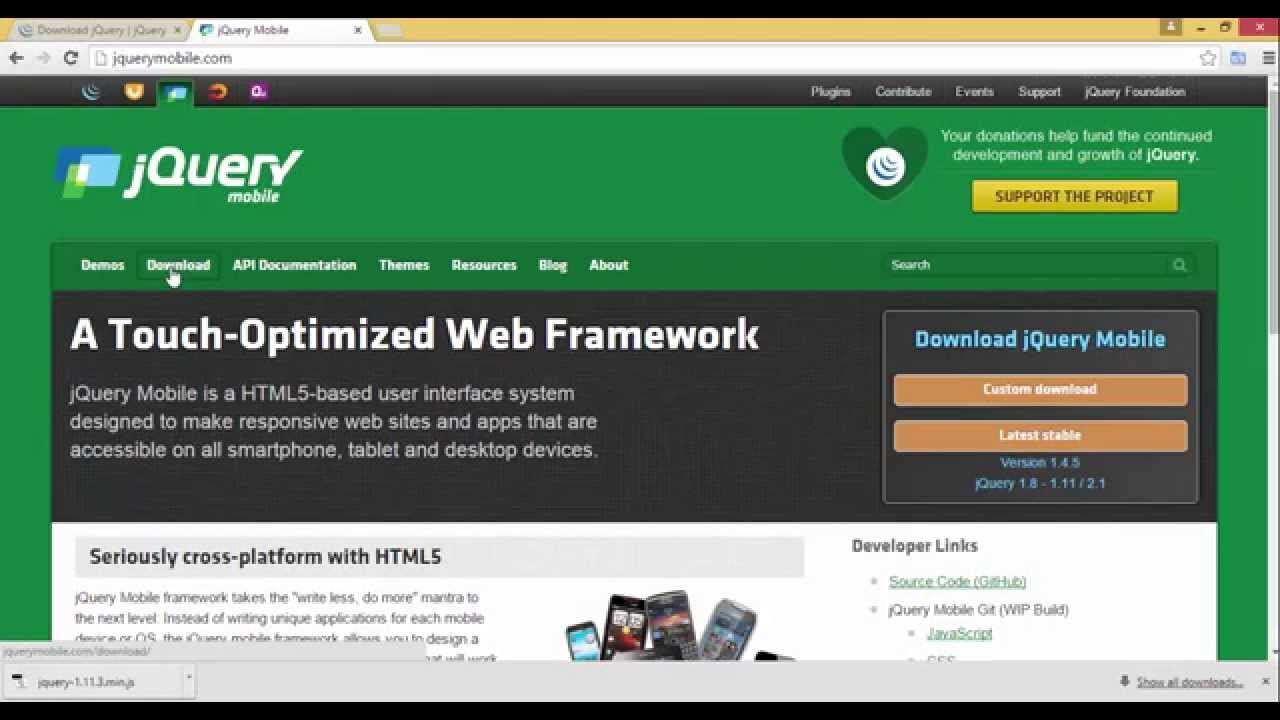Here is the cleaned-up version of the descriptive caption:

---

This image is a screenshot taken from a computer displaying the webpage for jQuery Mobile (jquerymobile.com). At the very top, occupying the upper 5% of the screen and set against a yellow background, there are tabs labeled "Download jQuery," "jQuery," and "jQuery Mobile." To the right, icons for profile management, minimizing, maximizing, and closing the window (with the 'X' icon notably in red) are visible.

Directly below this section, the primary navigation bar is displayed with the text "jquerymobile.com" prominently featured. Beneath this main navigation, another secondary navigation bar includes colorful icons on the left—blue, yellow, blue, orange, and purple. To the right of these icons are the hard-to-read navigation items, followed by clearer links labeled "Contribute," "Events," "Support," and "jQuery Foundation."

Moving further down, on the left side, there is the jQuery Mobile icon depicted with three rectangular boxes. Adjacent to the right, there is a dark green heart symbol resembling the Spotify logo, next to a statement that reads, "Your donations help fund the continued development and growth of jQuery." Below this statement is a gold-colored box with black text, "Support the Project."

Continuing down, there are various options listed: "Demos," "Download," "API Documentation," "Themes," "Resources," "Blog," and "About." On the left side of this list is a search bar.

Further down, the text reads, "A Touch-Optimized Web Framework," followed by additional details. To the right, buttons marked "Download jQuery Mobile" in orange and "Custom Download" labeled as "Latest, Stable" are visible. Below this section, another heading states "Seriously Cross-Platform with HTML5," followed by a descriptive paragraph.

---